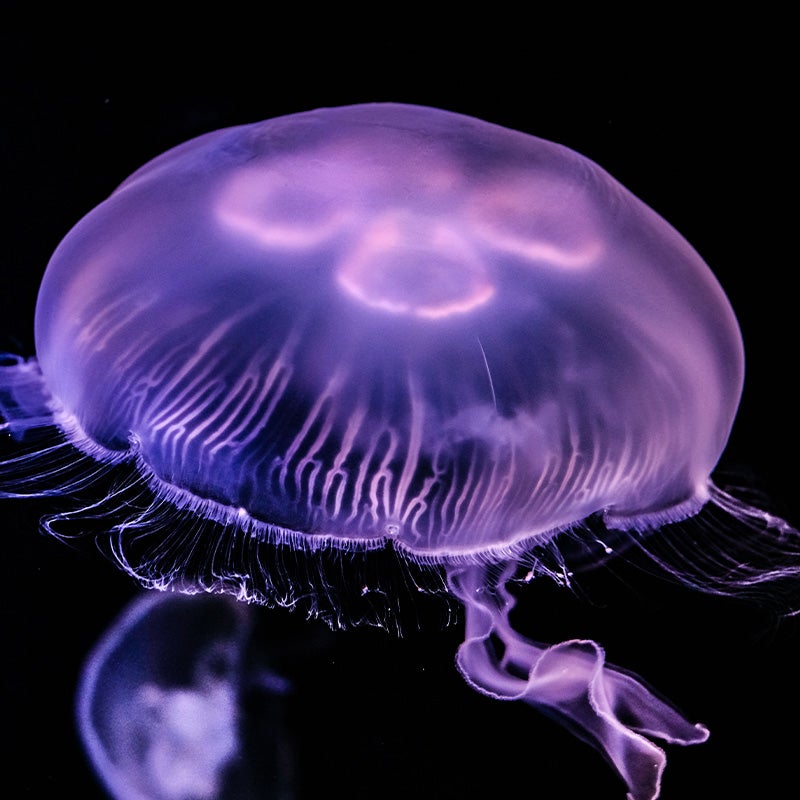This photograph captures a glowing jellyfish, its translucent, dome-shaped head brilliantly illuminated in a vibrant, grape purple hue. Viewed from a top-down angle, the jellyfish appears to be suspended in complete darkness, accentuating its ethereal glow against the solid black background. The dome-like body of the jellyfish reveals an intricate internal structure with hazy, frosted details, including four central orbs. Strands of delicate tentacles, wavy and fringed, cascade downward in varying shades of purple, adding to the enchanting, otherworldly atmosphere of the image. The overall composition is meticulously framed in a square format to highlight the jellyfish's luminescent beauty amidst the dark abyss.